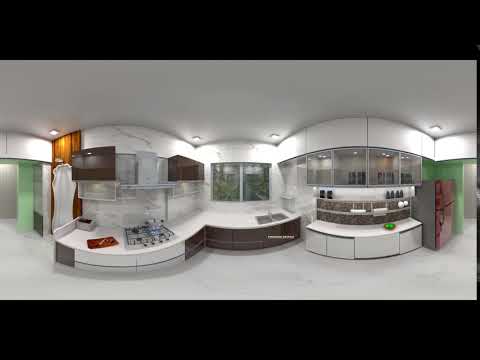The image presents a bright, expansive kitchen within a large room, featuring a pristine color palette dominated by white. The ceiling and walls are white, while the room is illuminated by recessed lighting fixtures, including four square lights. The kitchen is elegantly designed with intricate curves, giving it a modern look.

Two green doors are positioned on opposite sides of the room. On the left side, the kitchen begins with wooden cabinets and a gas stovetop featuring black cast-iron burners. Moving right, there is counter space with a large silver sink, which has double basins and sits beneath two expansive windows, allowing natural light to flood the room.

On the right side of the kitchen, there are additional countertops and cabinets. Some sections, including the upper cabinets, are made of glass, providing a glimpse of their contents. A striking brown section of cabinetry stands out amidst the primarily white decor. Adjacent to a green wall, a vibrant red refrigerator adds a pop of color. Additionally, the kitchen features a microwave hood.

A notable design element is the stone wall behind one of the countertop sections, adding texture and contrast to the sleek white surfaces and glass elements.